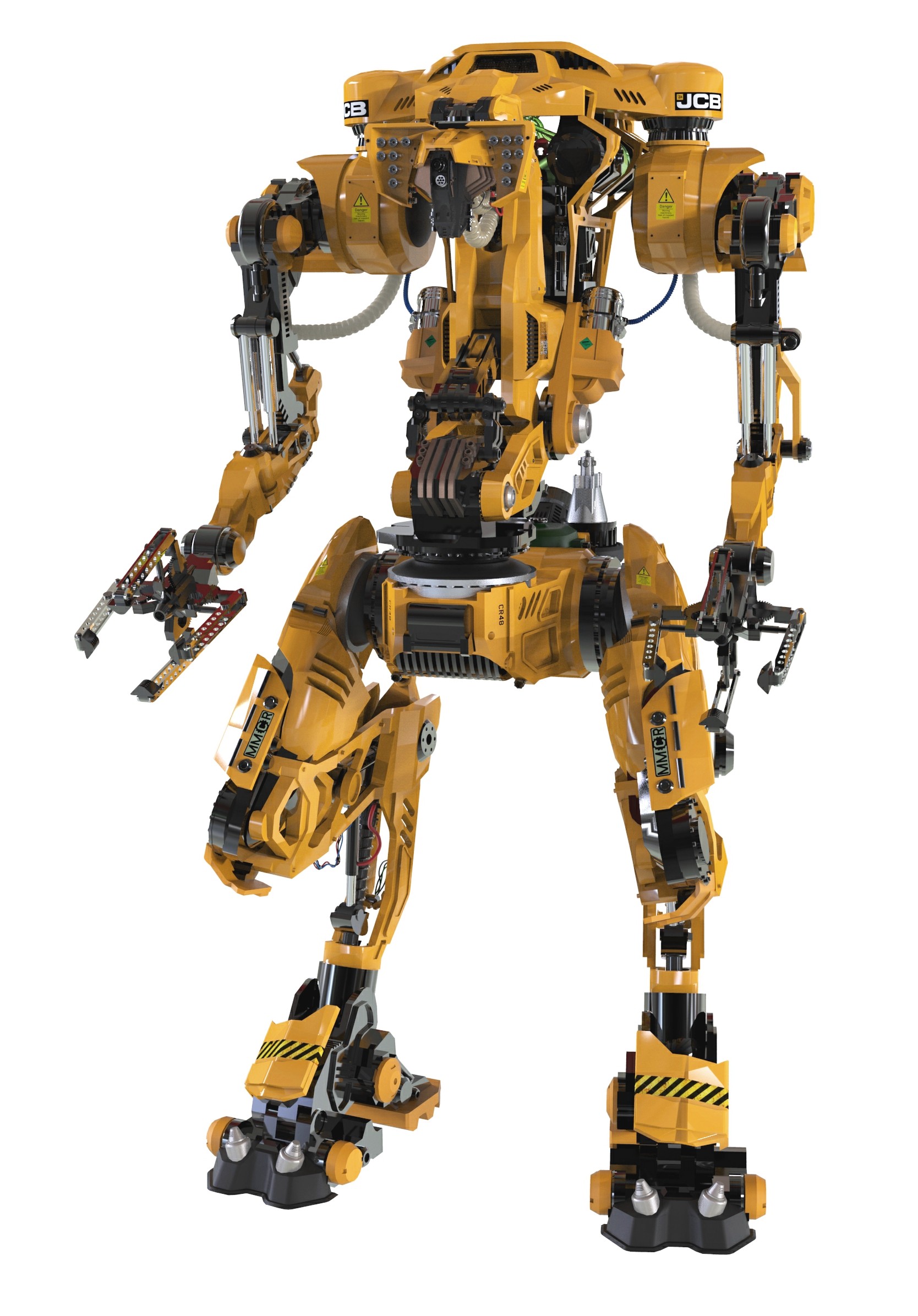The image showcases a computer-generated robot, predominantly colored in yellow with black highlights and some silver mechanical parts. Standing on two thick, V-shaped feet, the robot's legs are marked with the initials "JCB" and "MMCR." Its design is anthropomorphic, including a middle torso and wide shoulders from which its silver and yellow arms extend, ending in claw-like hands with four graspers arranged almost in a cube shape for versatile gripping. The head of the robot is flat and somewhat resembles a car viewed from the side, complete with sensors mimicking human facial features to provide a humanized appearance. The entire structure, set against a plain white background, gives it a simplistic yet magnificent look, reminiscent of Boston Dynamics' robots from a few years ago.